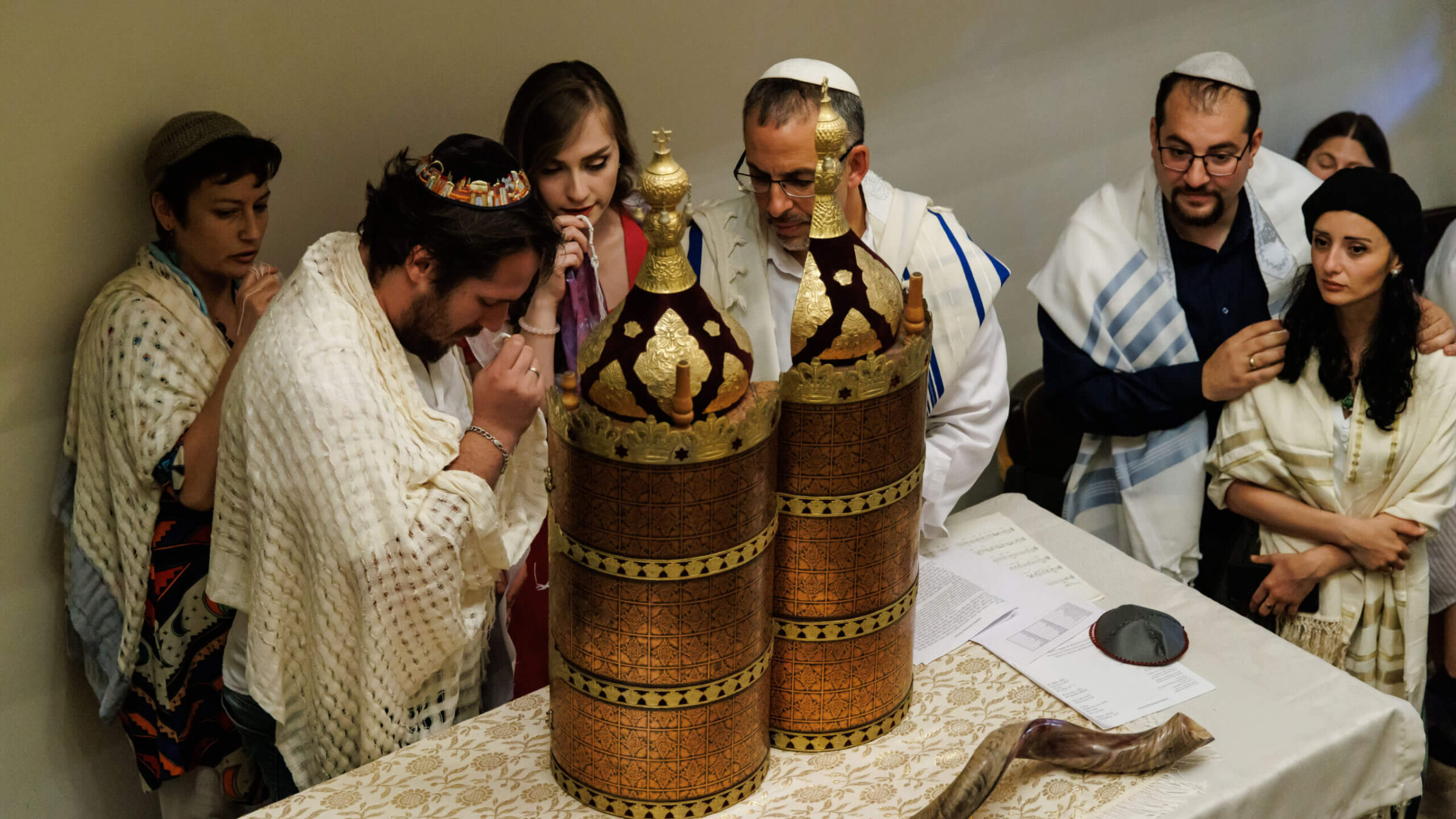The photograph captures a detailed and intimate scene of a Jewish religious ceremony or gathering, set indoors against a light brown wall. Central to the image is a long, rectangular table draped with a white tablecloth and a gold-and-white patterned runner. On the right side of the table, there are scattered papers.

At the center of the table stand two tall, cylindrical objects that are gold and bronze in color, each topped with steeples that have crosses at the tips. These are likely Torah scroll holders. Surrounding the table and praying are eight people: three men and two women on the left side, and one man and two women on the right side. The men are wearing yarmulkes, while all the participants have prayer shawls (tallit) draped around their shoulders. 

The individuals appear middle-aged, with dark hair, and are deeply engaged in prayer. One man, positioned centrally in front of the objects, appears to take on a leading role, similar to that of a priest or rabbi. The atmosphere is reverent, emphasizing the shared experience of faith and community.